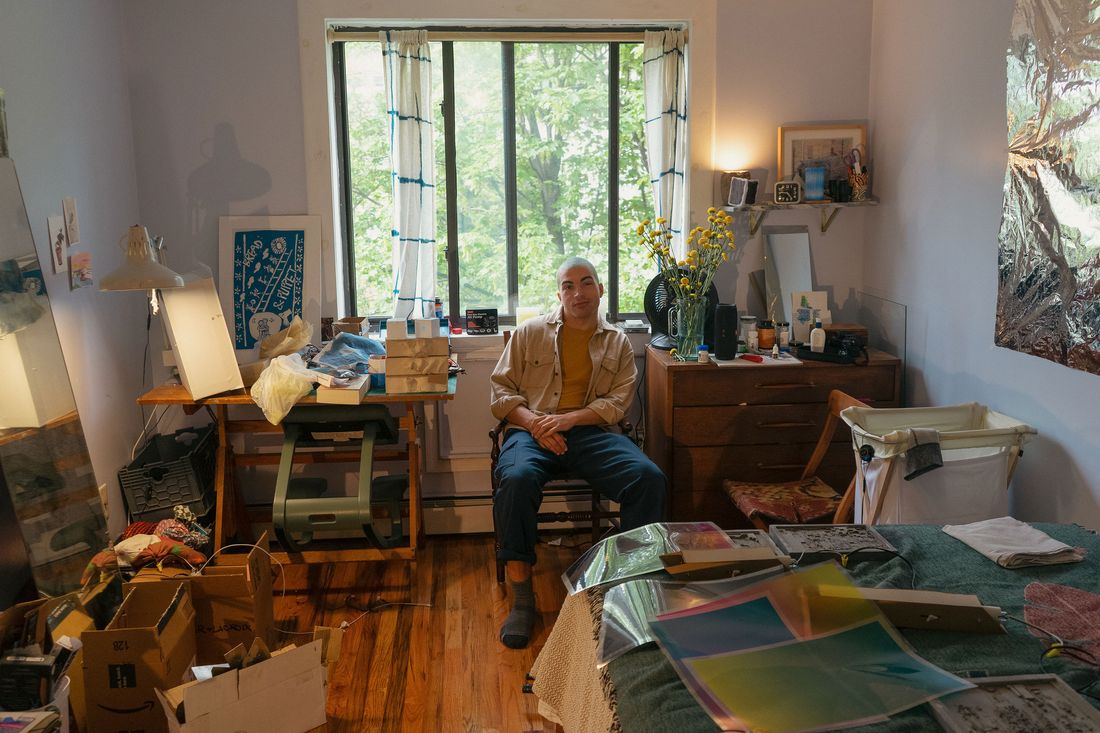In this color photograph, a bald-headed man is seated in the center of a cluttered bedroom, wearing an open, beige button-down shirt, blue jeans, and dark socks. He is sitting on a wooden chair with an open window behind him, through which green leaves and trees are visible, flanked by white curtains adorned with blue stripes. To his left, a desk brims with various items, including a white lamp, while boxes, including an Amazon box, sit on the wooden floor further left. To his right stands a brown bureau topped with yellow flowers in a vase, and assorted bottles. Above the bureau, a shelf holds more objects, including a clock, and a wall-hanging graces the upper right corner. Below, there appears to be a canvas laundry basket. In the lower right, a bed covered with a patch quilt is strewn with photographs, albums, a folded towel, and other items.